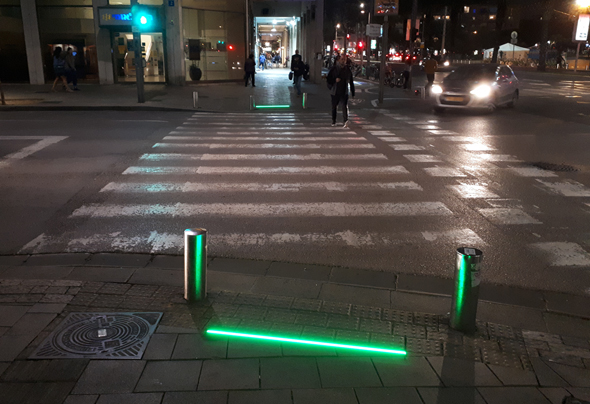This nighttime city street scene captures a bustling urban environment illuminated by the vibrant glow of streetlights and neon signs. The wide, well-marked crosswalk with horizontal striping is prominently featured in the foreground, where a circular iron sewer grate is also visible. A person dressed in black is walking towards the photographer from the far end of the crosswalk, while a car is in the process of making a right turn, likely stopping for the pedestrian. The distinctive green glow of a neon light, reminiscent of a "glow in the dark" stick or a "laser like they used in Star Wars," emanates from a fixture on the sidewalk. This light is positioned between two metal poles, casting an iridescent reflection on them. A traffic light aids in safely guiding pedestrians across the street. City lights from surrounding buildings and various other road markings can also be seen, enhancing the metropolitan ambiance of this vibrant, bustling street scene.